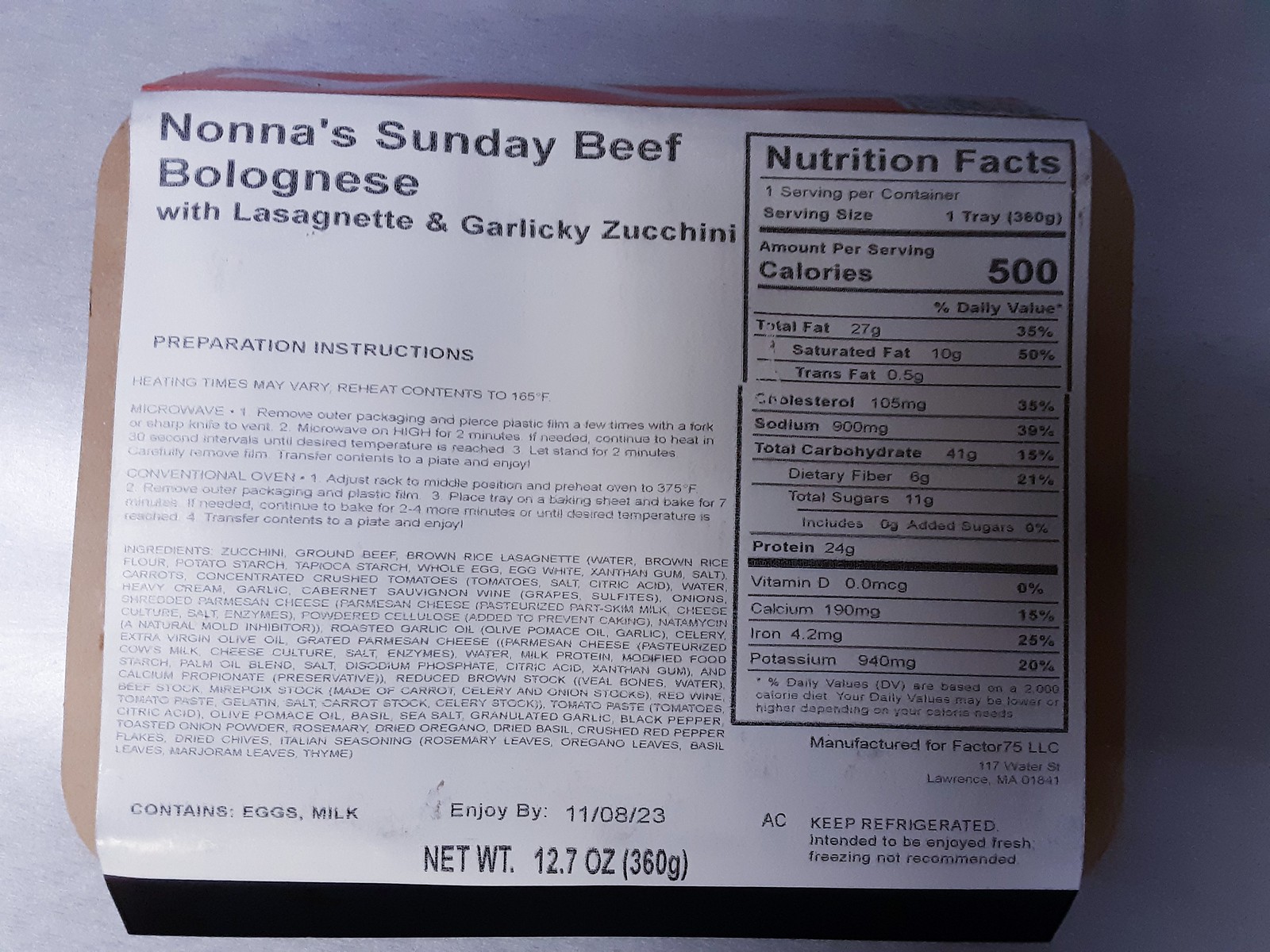This image features a photograph of a package label for "Nana's Sunday Beef Bolognese with Lasagna and Garlicky Zucchini." The label prominently displays the product title in the upper right corner. Below the title, extensive preparation instructions are provided, including guidance on varying heating times, pre-heating conditions, and ensuring the contents reach 185 degrees Fahrenheit. The instructions cater to both microwave and conventional oven methods. Beneath these instructions, a detailed list of ingredients is presented. Adjacent to the preparation guidelines, on the right side of the label, is the nutrition facts panel. The package is set atop a gray or silver tabletop, adding a subtle backdrop to the scene.